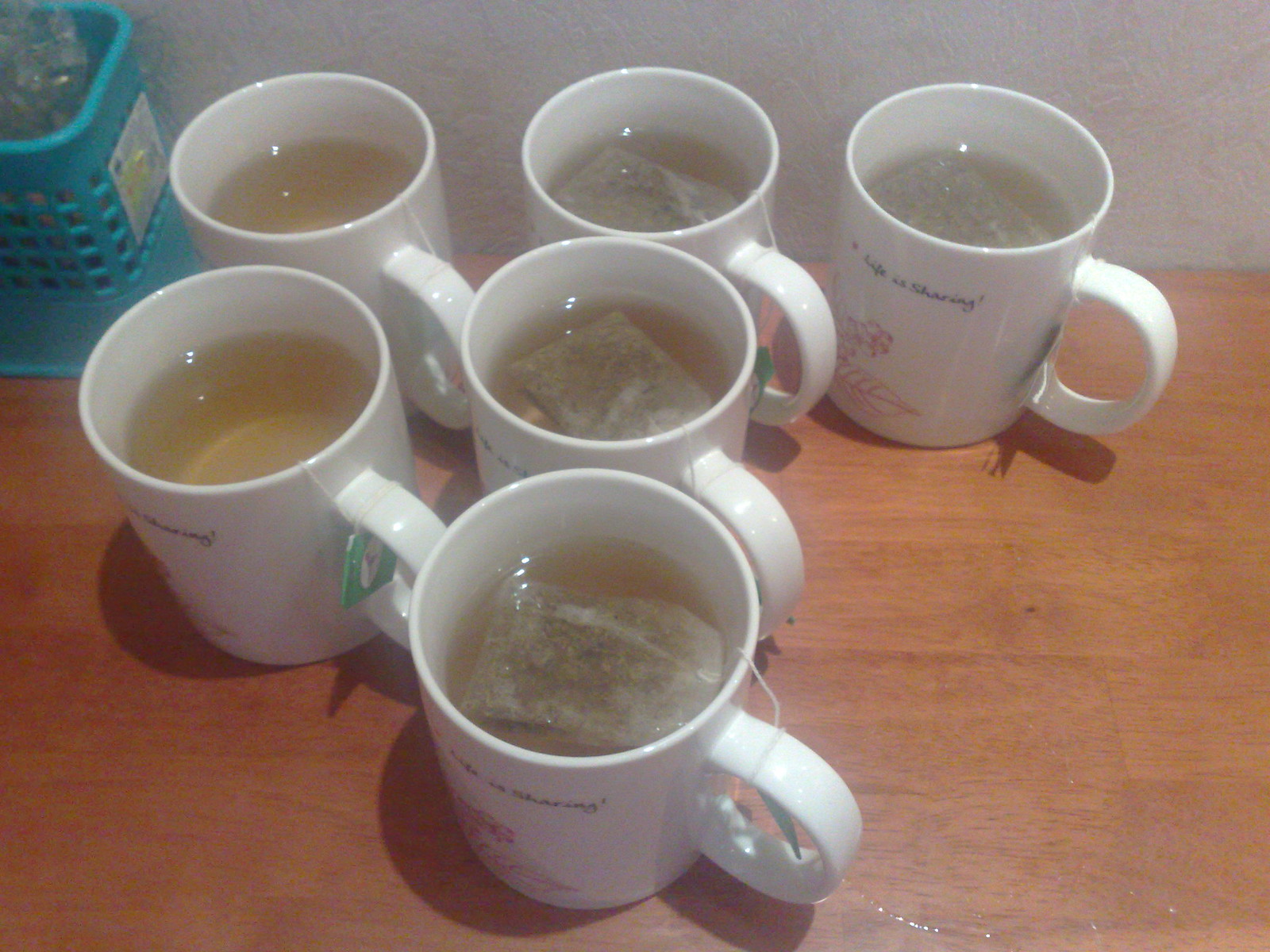This is a slightly out-of-focus photograph of six identical white mugs positioned on an oak-colored wooden table. Each mug features a white handle and is adorned with a delicate pink and red floral design, accompanied by cursive black text reading "Life is Sharing." The mugs are filled with a clear brown liquid, indicating tea, with strings from the tea bags visible hanging out the sides. Four of the six mugs have tea bags floating on the surface, while the other two have the tea bags submerged. A blue container with holes is situated to the left of the mugs. The setting includes shadows around the cups, suggesting it is a well-lit room, and a white wall can be seen in the background. The photo is taken from a top-down perspective, giving a clear view into the mugs.